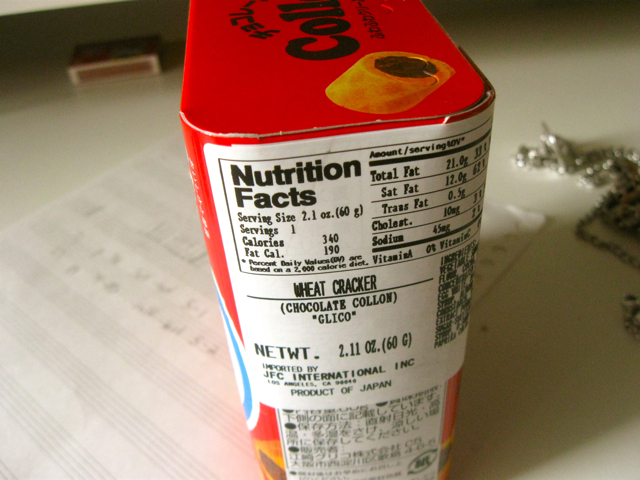This is a photograph of a red canister-shaped container of snack food, prominently displaying a white nutrition label. The label details serving size, calories, fat calories, total fat, saturated fat, trans fat, cholesterol, sodium, vitamin A, and vitamin C. The product is identified as a wheat cracker with a chocolate filling, imported by JFC International in Los Angeles, and is a product of Japan. The container also mentions "colonne" or "calo," likely indicating the type of snack. It is sitting on a white table, atop a sheet of musical notation, with a pencil resting on it as if someone were writing a song. Beside the container are a box of matches and a gold chain necklace. Additionally, there are some elements not fully visible, including a blue circular shape and several ingredients listed on the side of the canister, which are not clear in the photograph.